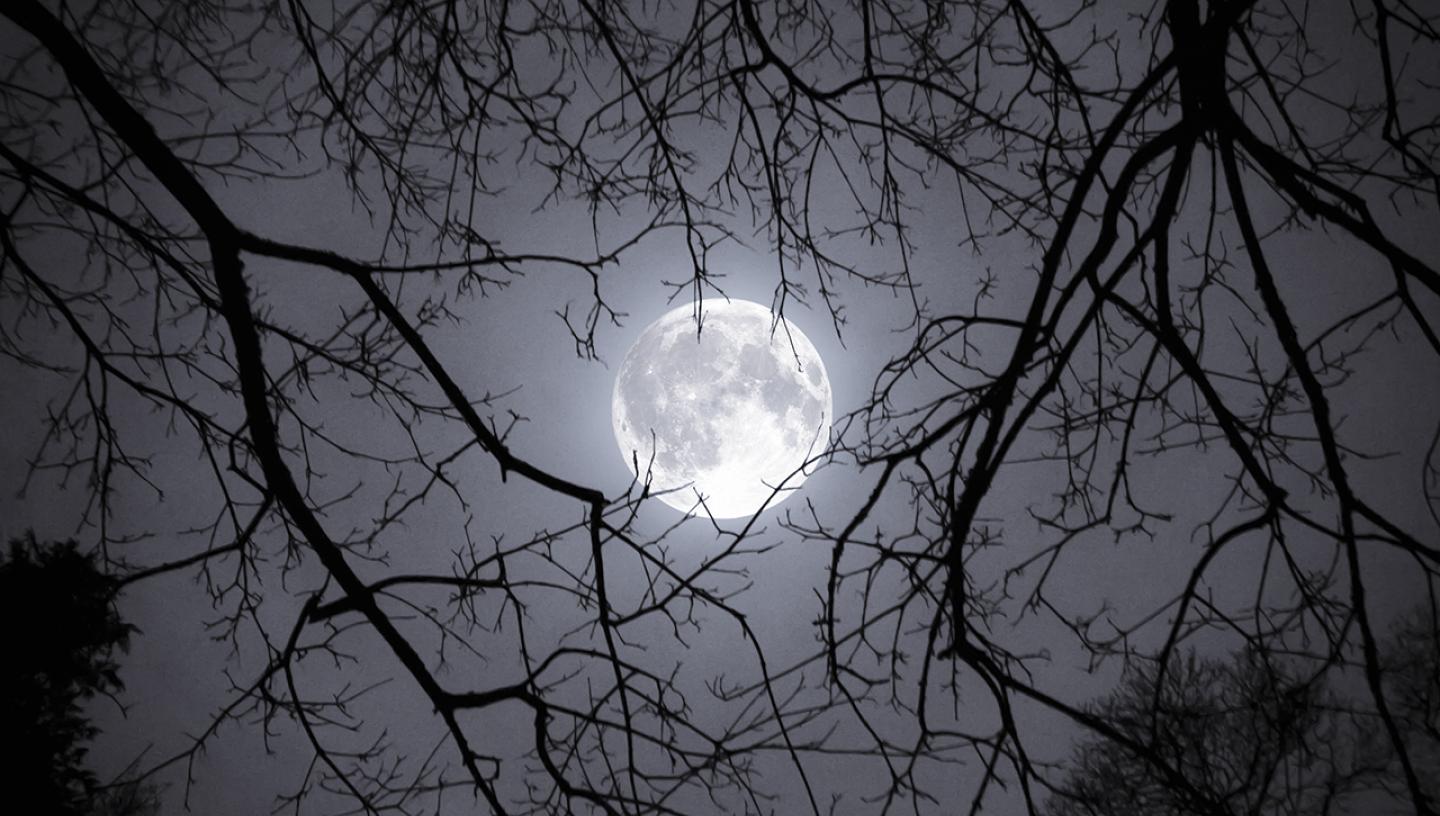The photograph captures the glowing white full moon, centered amidst a vast night sky devoid of stars. The sky appears as a gradient of light gray, with a semi-transparent halo of moonlight surrounding the moon, and darkens towards the edges. The moon itself showcases various gray craters and markings, adding texture to its luminous surface. 

Bare black tree branches frame the scene, their starkness accentuated by the poor lighting, making them appear almost as shadows. The branches intrude subtly into the moon's space, particularly from the top and top right, where a large branch arches down with numerous offshoots. Additional branches from the bottom left and bottom right corners contribute to the intricate latticework.

In the bottom left corner, a fuller tree with remaining leaves casts a dark silhouette, while a distant, bare tree stands in the bottom right, shrouded in the same eerie moonlit ambiance. The overall composition is rectangular, with the top and bottom sides twice the length of the left and right sides, creating a panoramic view of this moonlit night through a veil of skeletal branches.